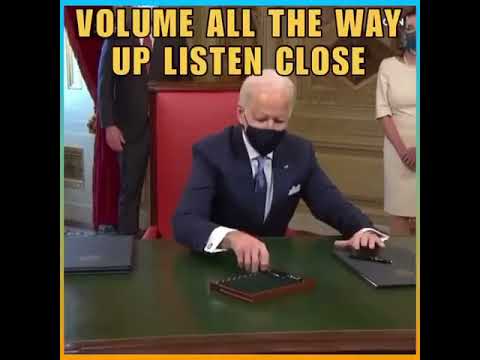The image is a wide rectangular frame primarily featuring black sections on the left and right edges. In the center is a square meme of President Joe Biden at his desk in the White House. The desk has a green surface with brown wooden borders, and on it are several free notebooks and a couple of pens. President Biden, wearing a black face mask, a blue suit, a light blue collared shirt, and a blue tie, is sitting in a tall chair made of dark brown wood with a red velvet back. He is holding a pen with his right hand hovering over what appears to be a gray metal folder or possibly a laptop.

To his right stands a woman in a white dress and mask, her arms held in front of her. Behind Biden's red velvet chair, there is another man standing, dressed in a suit, and partially visible due to their positioning. The background indicates they are in a room in the White House, possibly with a large curtain behind them. Surrounding the meme is a gradient border transitioning from light blue at the top, to green in the center, and merging into yellow and orange at the bottom. The top of the image contains text in yellow and orange that reads, "Volume all the way up, listen close."